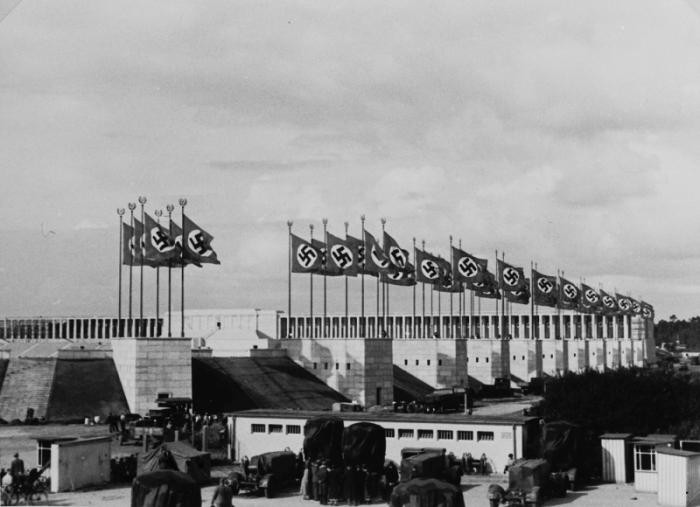This black-and-white photograph captures an extensive row of long, rectangular, mostly featureless gray stone buildings, reminiscent of mid-20th century Nazi architecture, possibly from World War II or the 1930s. Each building in the row has a single line of windows on the second floor and a door at each end. Protruding edifice structures with a total of 66 flagpoles are evenly spaced along the buildings, each flying a distinct red Nazi flag adorned with a white circle and black swastika. In front of these main buildings, there is a lower, elongated structure, and parked in the foreground are several mid-20th century military trucks, covered with tarps. The cloudy sky adds to the somber atmosphere, while a few individuals appear to be standing near the vehicles, possibly part of a military outpost.